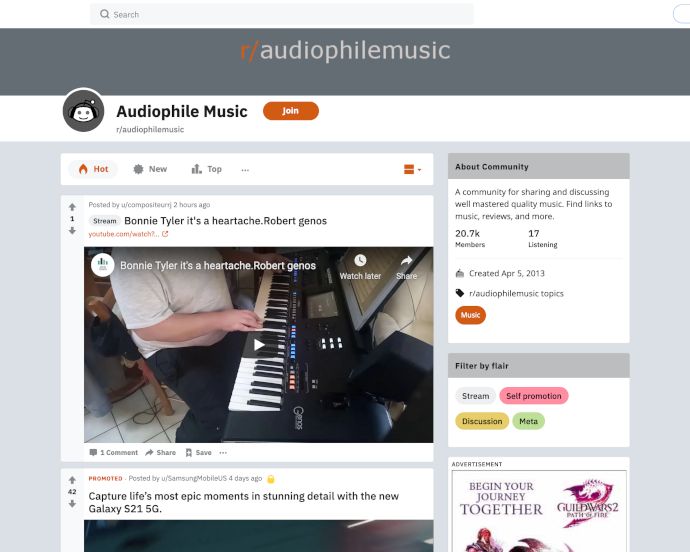The image depicts the homepage of a website called "Audiophile Music." At the top, there is a slim search bar centered on the page. Directly below the search bar is a grey banner featuring the website's name, "Audiophile Music," prominently in the center. Beneath this banner, there is a circular logo representing the website and an orange "Join" button positioned to the right.

The main section of the site has a grey background and includes navigational tabs labeled "Hot," "New," "Top," and more. In the featured content area, there is a video thumbnail displaying someone playing a keyboard. The video is of Bonnie Tyler's song "It's A Heartache," and it has a play button that users can click to watch. The video has attracted three comments so far.

On the right-hand side of the page, an "About Community" section provides additional information, noting that the community has 20.7 thousand members and that 17 people are currently active on the forum. Further down, the page offers various filter options and features an advertisement occupying part of the front page real estate.